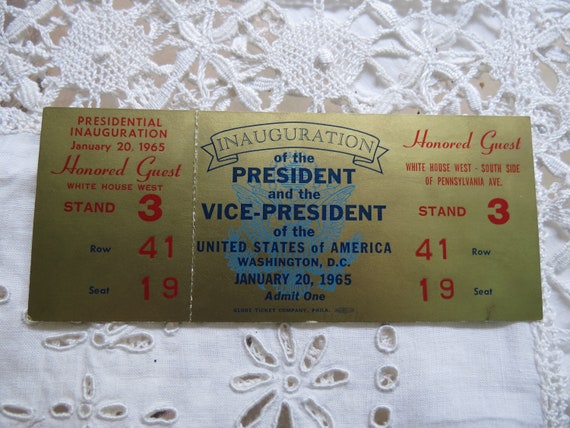This photograph captures an unused, golden-hued ticket from the presidential inauguration on January 20, 1965, placed on a white lace tablecloth. In the center, the ticket displays in blue lettering: "Inauguration of the President and the Vice President of the United States of America, Washington, D.C., January 20, 1965. Admit One." To the right, "Honored Guest, White House West, South Side of Pennsylvania Avenue, Stand 3, Row 41, Seat 19" is printed in red letters. The left side of the ticket, still intact, is perforated for detachment and repeats the information: "Presidential Inauguration, January 20, 1965, Honored Guest, White House West, Stand 3, Row 41, Seat 19." The ticket was issued by the Globe Ticket Company.